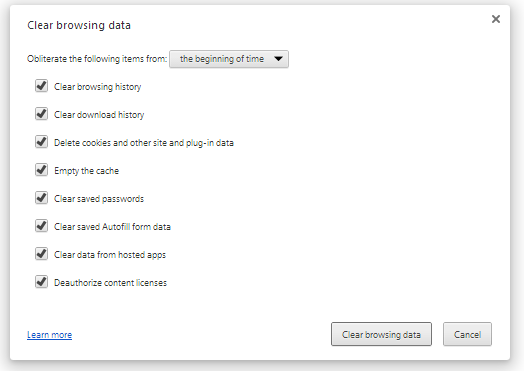The image displays a detailed view of a browser's "Clear Browsing Data" dialog box. 

The main section of the box is white with a light gray border. In the top left corner, the text "Clear browsing data" is prominently displayed, while a small "X" icon is situated in the top right corner, indicating the option to close the dialog.

Below this header, the text "Obliterate the following items from:" appears, accompanied by a drop-down menu set to "the beginning of time." This implies that the clearing actions will affect all data from the start of the browser's history.

In the subsequent section, a series of checkboxes are aligned along the left side, all of which are checked. The options listed from top to bottom include:
- Clear browsing history
- Clear download history
- Delete cookies and other site and plug-in data
- Empty the cache
- Clear saved passwords
- Clear saved Autofill form data
- Clear data from hosted apps
- Deauthorize content licenses

Below these options, a blue hyperlink labeled "Learn more" offers additional information regarding the action.

Towards the bottom right of the dialog, there are two horizontal buttons. The larger button, with a white background and black border, contains the text "Clear browsing data" in gray. Adjacent to it, there is a smaller, similarly styled button that reads "Cancel," providing an option to abort the action.

This detailed depiction ensures a comprehensive understanding of the browser's data clearing interface.